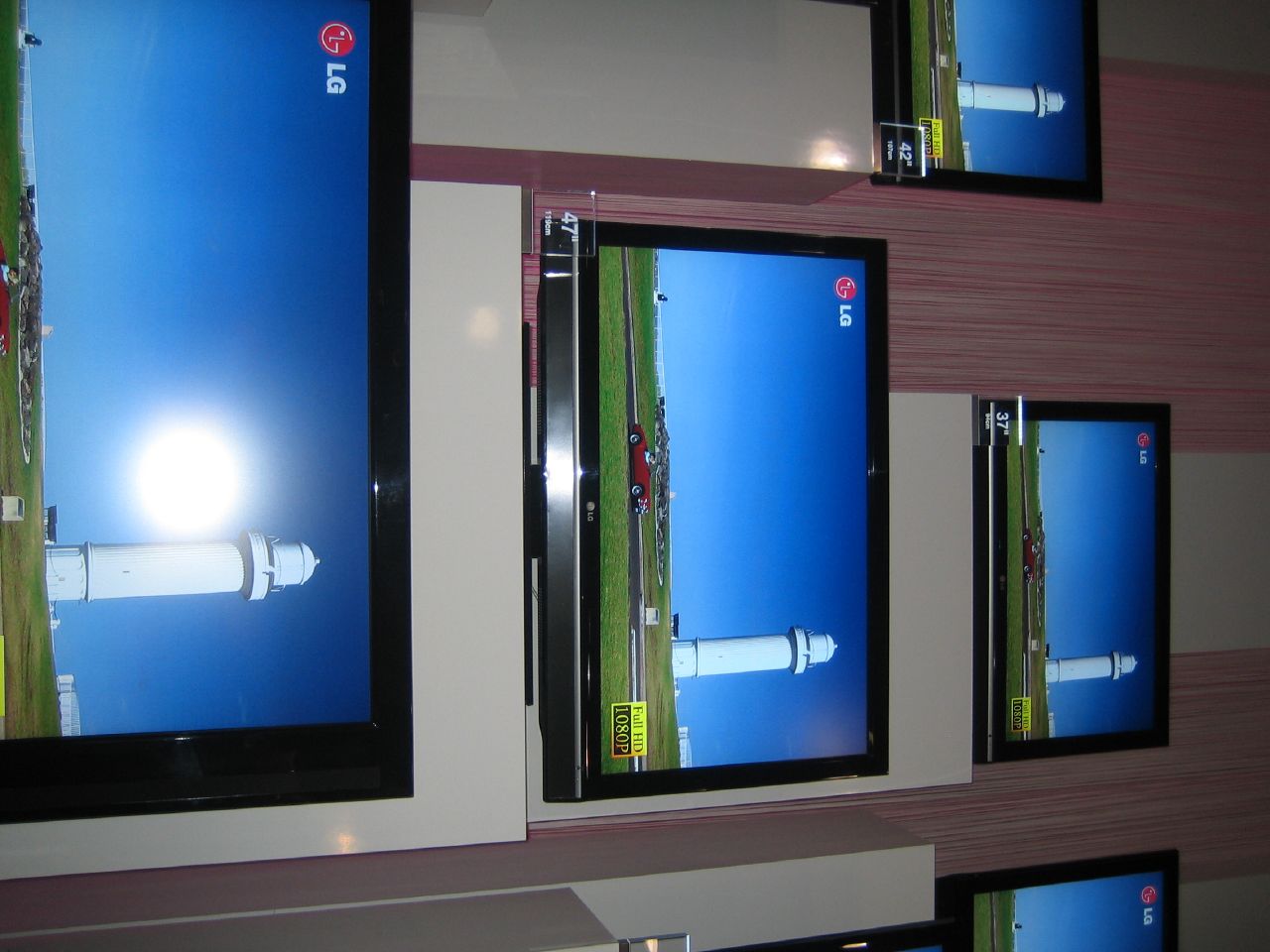This detailed color photograph depicts a retail store display featuring five LG monitors of different sizes, neatly arranged on individual pedestal-type risers against a backdrop of grayish tan and burgundy-striped faux wood wallpaper. The largest monitor, a 47-inch screen at the center bottom, suffers from a camera flash reflection near the middle, directly to the left of a large white, tower-like structure, presumably a lighthouse. The image on all screens shows a scenic landscape with a red sports car poised on a green, grassy field under a blue sky, prominently featuring a tall white lighthouse. Each monitor prominently displays the LG logo in the upper left corner, with additional text indicating "Full HD, 1080p" and specific screen sizes including a 27-inch monitor at the top center and edges showing partial views of 42-inch and 37-inch screens to the left and right, respectively. The detailed setup and uniformity of the displayed image suggest this is a section of an electronics store dedicated to showcasing LG's flat-screen monitors.